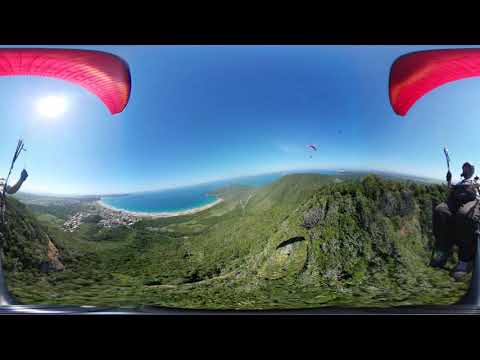This highly detailed outdoor image captures a 360-degree view of a man parachuting over a scenic landscape. The parachute, which is distinctly red, arches above him, with its connecting wires visible on both sides of the frame. The man, equipped with a helmet, dark attire, and copper shoes, is in a seated position, grasping the parachute straps as he descends. The scene unfolds against a vivid blue sky, accented by the sun on the left. Below, the terrain features a green, mountainous island with lush cliffs and foliage, bordered by the shimmering ocean. The horizon reveals another parachuter in the distance. The image's distortion creates an expansive, all-encompassing view of the picturesque landscape, combining elements of water, greenery, and a small shoreline town, giving an immersive feel of the thrilling descent.